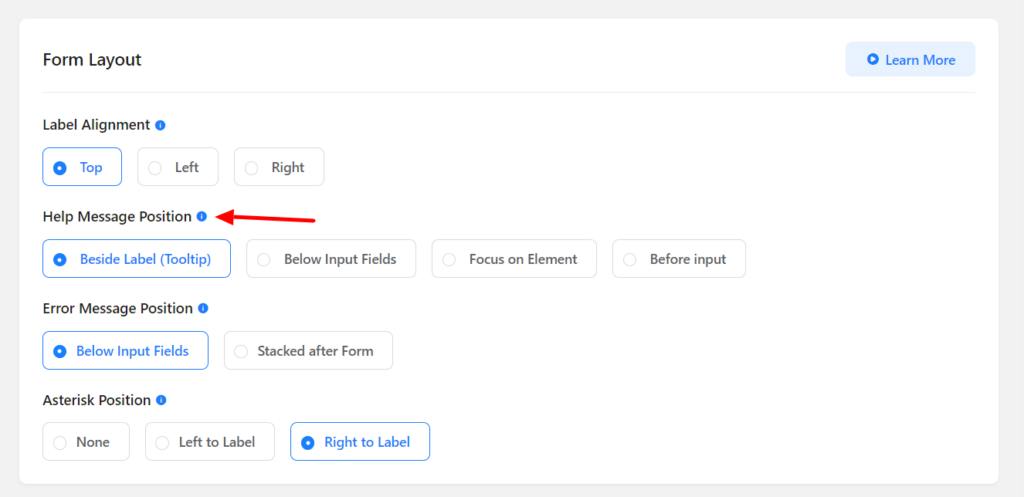This image is a screenshot of a form on a website, featuring a muted gray thick border encasing a white window. In the top left corner, the text "Form Layout" is displayed in black. On the upper right side, a light blue bar contains a circular blue icon with a white arrow pointing to the right and the text "Learn More" written in blue.

Beneath "Form Layout," the section labelled "Label Alignment" appears on the left-hand side, accompanied by a blue information bubble to its right. There are three radio button options below this label: 
- The first option, "Top," is highlighted in blue, indicating it is selected.
- The second option, "Left," is gray.
- The third option, "Right," is also gray.

The next line features bold black text "Help Message Position," with a blue information bubble to its right. A long red arrow points directly to this information bubble. Under this section, there are four radio button options:
- The first option, "Beside Label Tooltip," is selected and thus appears in blue.
- The second option, "Below Input Fields," is gray.
- The third option, "Focus on Element," is gray.
- The fourth option, "Before Input," is also gray.

Continuing, the next bolded black section titled "Error Message Position" has a blue information bubble to its right. It includes two options:
- The first option, "Below Input Fields," is selected and appears in blue.
- The second option, "Stacked After Form," is gray.

The final section is titled "Asterisk Position," with a blue information bubble on its right. This section contains three radio button options:
- The first option, "None," is gray and not selected.
- The second option, "Left to Label," is gray.
- The third option, "Right to Label," is selected and appears in blue.

Overall, the form's layout demonstrates various user settings, providing options for label alignment, help message positioning, error message positioning, and asterisk positioning, each supported with clear visual indications and explanatory tooltips.